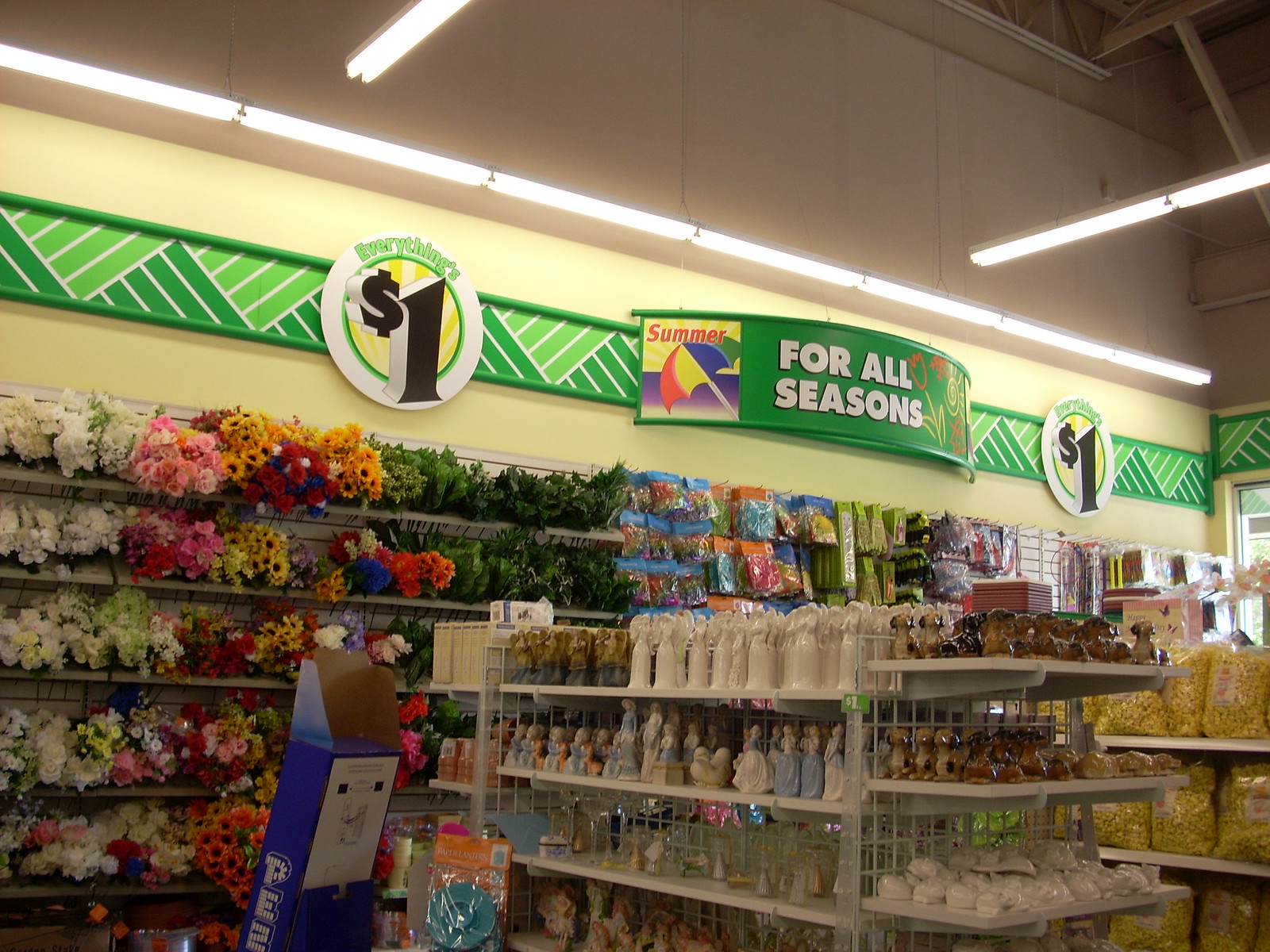The photograph depicts the interior of a discount dollar store featuring a high, A-frame ceiling with conspicuous rows of fluorescent lighting and a warehouse-like ambiance. The yellow walls are adorned with a green band near the top, accented with triangular patterns in varying shades of green. Prominently displayed on the wall is a large circular logo proclaiming "Everything's One Dollar," with an additional semi-circular sign stating "For All Seasons" and highlighting "Summer" with an umbrella graphic. The back wall is lined with shelves brimming with an assortment of artificial flowers including white sunflowers and a mix of pink and white blooms. In the foreground, white shelving units house an array of angelic figurines adorned in blue dresses, alongside other religious figures. Nearby, end caps feature seated dog figurines. A perpendicular shelf towards the background is stocked with bags of what appears to be popcorn. The scene captures the eclectic array of dollar-priced items under the store's signature fluorescent brilliance.